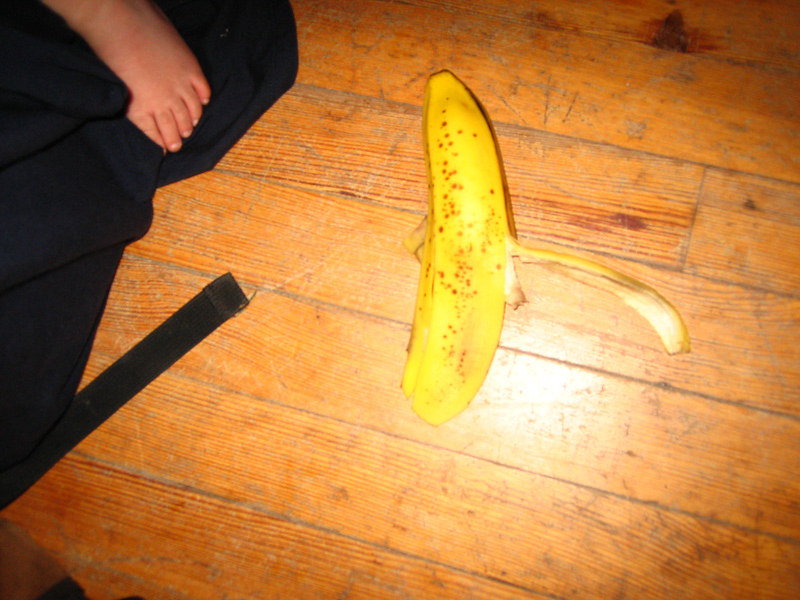A brightly lit, overexposed photograph captures an aged pine wood floor, its surface showing the accumulated residues of wax and embedded dirt within the grooves, creating a grayish-brown contrast. Centered near the top of the image lies an empty banana peel, its fruit possibly still hidden inside the unpeeled portion, though it's unclear. A prominent white reflection, likely from a camera flash, dominates the middle of the picture, further illuminating the scene. The wooden floorboards align in a downward slant from left to right. Towards the left side of the photograph, a partially visible foot, covered in a black cloth, reveals most of its toes but leaves the large toe obscured.